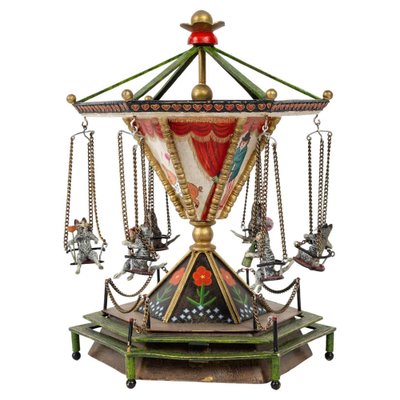This image features a highly detailed tabletop decoration resembling an antique 1800s amusement ride. The structure, likely crafted from tin and wood, mimics a carousel with tiny swings suspended by chains, each featuring an animal, possibly cats, holding flowers and seated in the chairs. The decoration stands on a base with a roughly hourglass shape and a hexagonal frame, detailed with six black panels adorned with red flowers on green stalks, accompanied by smaller white flowers. These panels taper towards a central golden ball and expand again towards the top, where six green bars rise to a decorative hexagon crowned with golden finials, a red half ball, and a golden flower. The overall color palette includes green, white, gold, black, red, blue, silver, and brass, with intricate floral designs highlighted at the base. The item is designed to spin, allowing the swings to flair outward, mimicking the motion of a classic carnival ride.